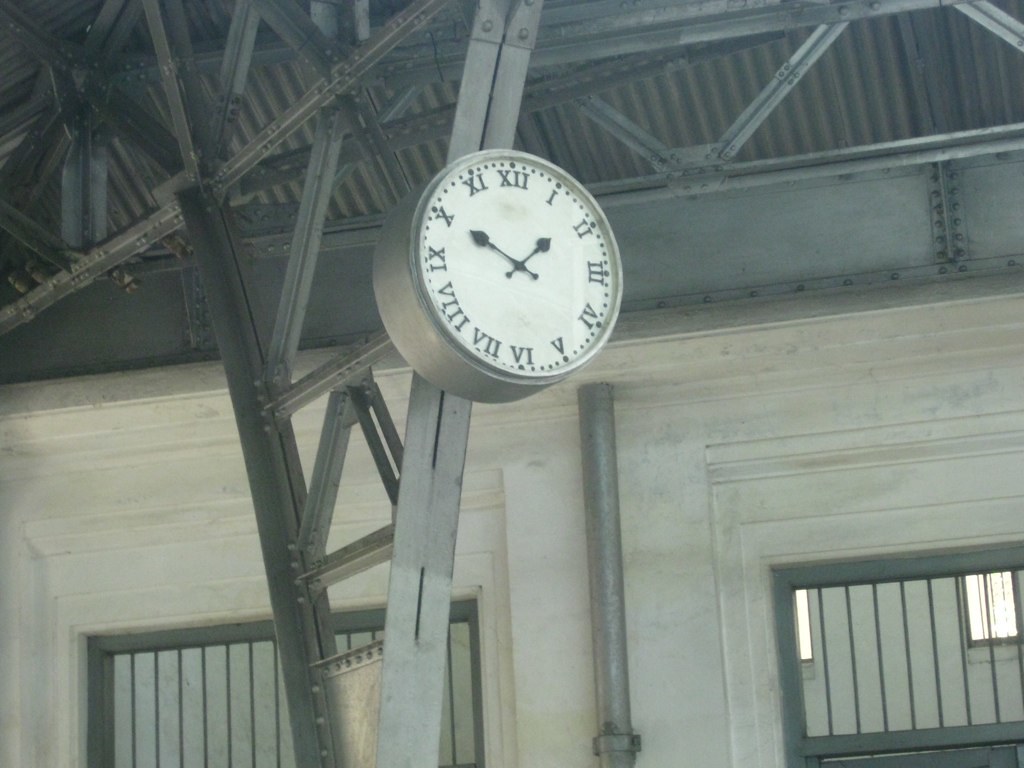This detailed, descriptive caption outlines what the image depicts:

"Although the image is greyscale, subtle yellowish tints give it an almost painting-like, non-photorealistic appearance. Centrally featured is a round clock face with a metallic edge, attached to a metal beam extending from the ceiling and reaching downward toward the floor. Behind the clock, a crooked metallic ladder or structure can be seen, adding to the industrial feel of the setting. The ceiling is comprised of galvanized metal beams, while the walls appear to be made of grey wood with windows framed by vertical bars. The clock face is stark white, marked by Roman numerals from I to XII, accompanied by small dots between the numerals. There are two black hands with rounded tips, currently indicating the time as approximately ten minutes past two."